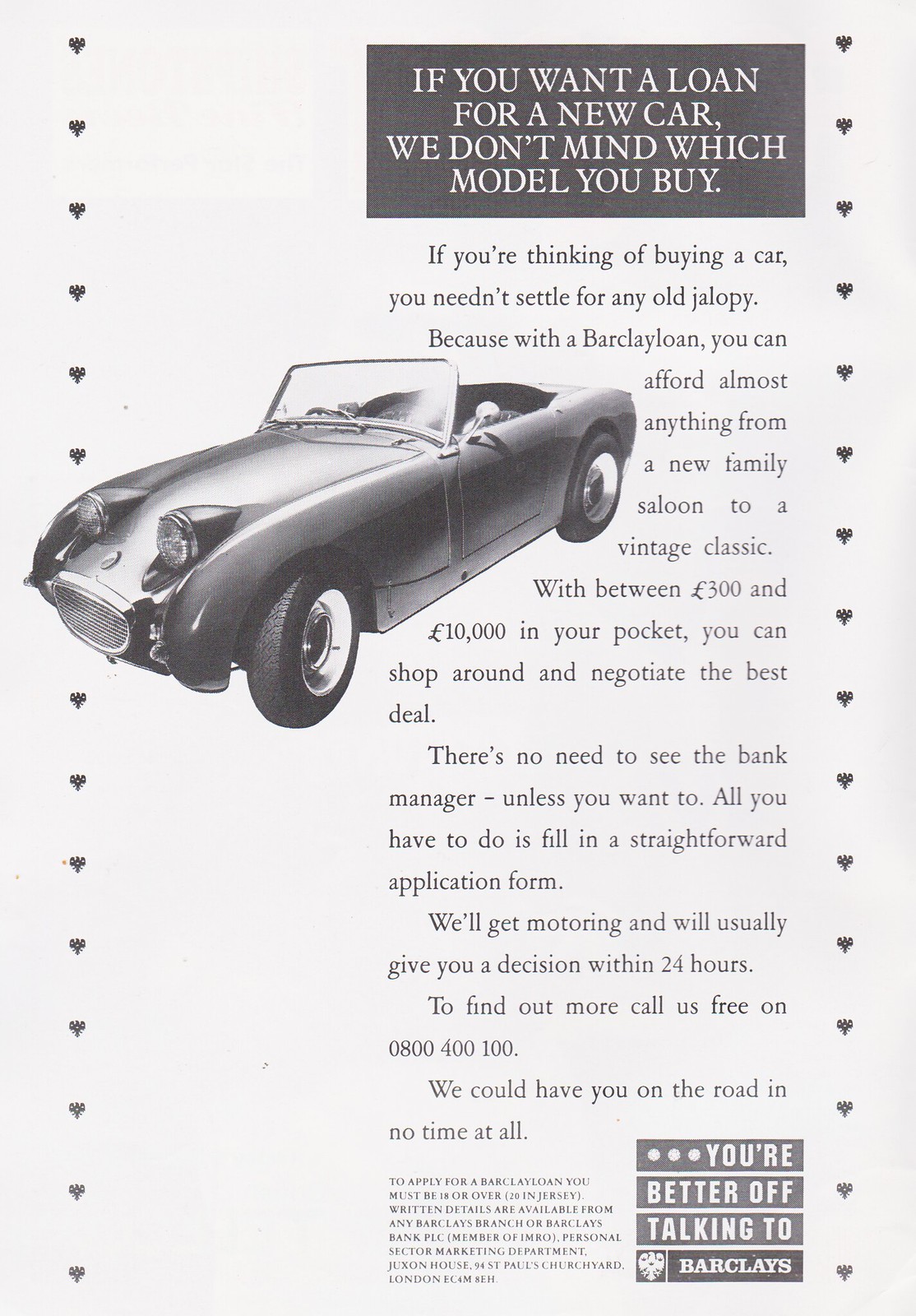This black and white magazine advertisement promotes Barclays' car loan services, featuring a vintage sports car prominently displayed on the left side of the image. The caption at the top right reads, "If you want a loan for a new car, we don't mind which model you buy." The advertisement encourages potential buyers not to settle for an old jalopy, highlighting that with a Barclays Loan, they can afford almost any car, whether it's a new family saloon or a vintage classic, with loan amounts ranging from $3,300 to $10,000. The process is described as simple, requiring only a straightforward application form without a mandatory visit to the bank manager. Barclays promises a decision within 24 hours, emphasizing their efficiency with the tagline, "We could have you on the road in no time at all." For more information, readers are invited to call 0800 400 100. At the bottom, alongside the Barclays logo, the ad reinforces its message with, "You're better off talking to Barclays."